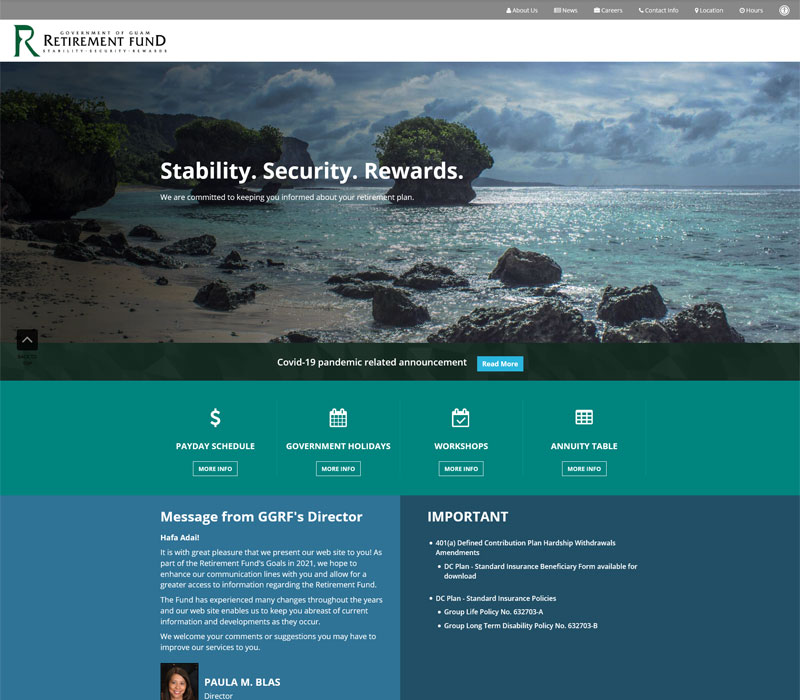The web page features a clean and modern layout with a well-organized structure. In the upper-right corner, there's a green capital "R" logo. Directly to the left of the logo is the title "Retirement Fund" in black text. Overlaying part of this title is some additional text, which is somewhat obstructed. Beneath the "Retirement Fund" text, there is a small, hard-to-read link. 

Below these elements is a horizontal navigation bar with six menu items, followed by an eye icon situated toward the right end of a gray title bar that overlaps with the "Retirement Fund" text/logo.

The main content of the web page highlights a promotional cover image featuring a calming sea and beach scenery. Overlaying this image is a bold, concise message: "Stability. Tech. Security. Rewards. We are committed to keeping you informed about your retirement plans." 

Additionally, there's a COVID-19 pandemic-related announcement with a "Read More" button, easily noticeable due to its green color. Further down, the page includes several highlighted sections such as "Payday Schedule," "Government Holidays," "Workshop," "Annuity Table," and "Message from GGRF's Director, Paula."

To the right of these sections, there is the word "Important," signaling crucial information or updates.